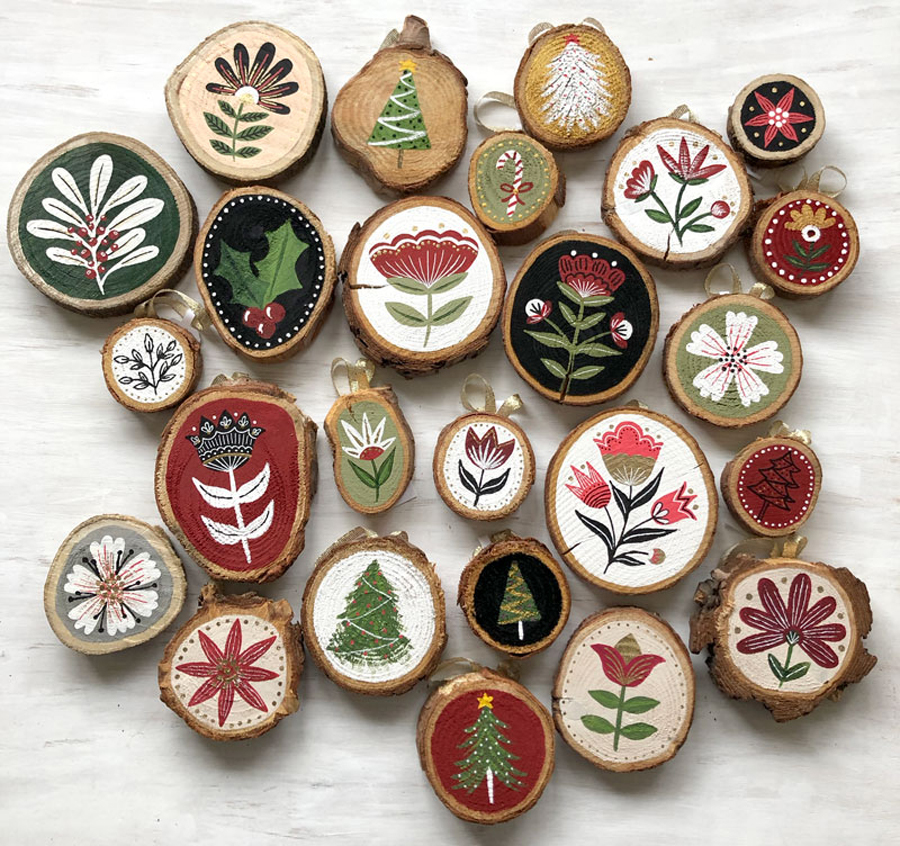The photograph features a square format showcasing an exquisite collection of handmade wooden ornaments, all centrally placed against a light ashen white marble-like background with grey streaks. This assemblage consists of round cross-sections of branches that vary in thickness, some retaining the texture of bark while others reveal the smooth, bark-less wood. The sizes range from small penny-like discs to larger drink coaster dimensions.

Each ornament is meticulously hand-painted, predominantly using acrylic paint, with designs reflecting Scandinavian or Pennsylvania Dutch motifs. The decorations are botanical and Christmas-themed, featuring stylized trees, flowers, holly with berries, poinsettias, mistletoe, and more. The color palette is rich and varied, with primary hues of green, red, black, and white, but also incorporating bursts of pink, gold, purple, and yellow.

One ornament, painted on a bare wood background, displays a Christmas tree adorned with a yellow top and a white garland zigzag, while another features a black background with white dots encircling its edge. A standout piece depicts a sprig of holly with two green leaves and three red cherries. Additional designs include white petals with orange streaks, and a Christmas tree with a yellow star on a red background. Elsewhere, a green background supports a candy cane with a ribbon, and yet another ornament showcases a poinsettia on a gray background.

In total, there are around 20 such detailed, painted wooden slices, each contributing to the festive and artisanal charm of the photograph.